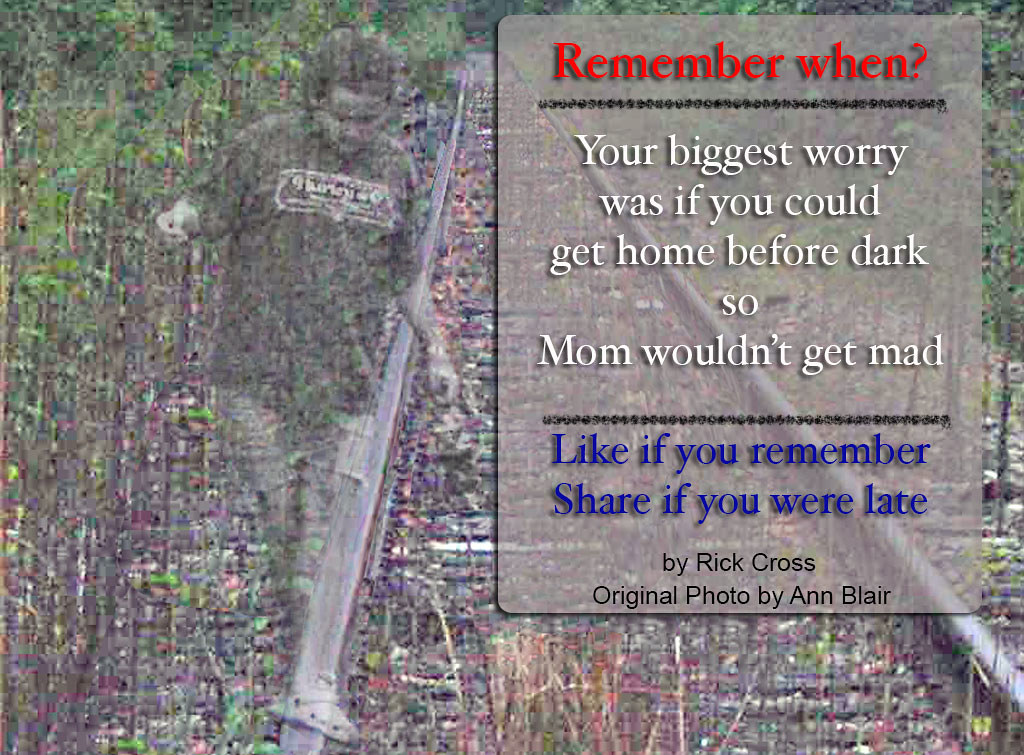This is a pixelated and monochromatic poster featuring a faded image of a teenager balancing on railroad tracks, dressed in shorts, a dark t-shirt, and sandals which appear to be Crocs. The scene, devoid of color and surrounded by tall grass, evokes a nostalgic mood. Overlaying the photo on the right side is a semi-transparent, gray rectangle containing text. The text starts with "Remember when" in red, followed by "your biggest worry was if you could get home before dark so mom wouldn't get mad" in white, and concludes with "Like if you remember, share if you were late" in blue. At the bottom, it credits Rick Cross and mentions that the original photo is by Ann Blair. The overall quality of the image is low, with noticeable colorful noise and transparency effects suggesting it might be a superimposed photo.